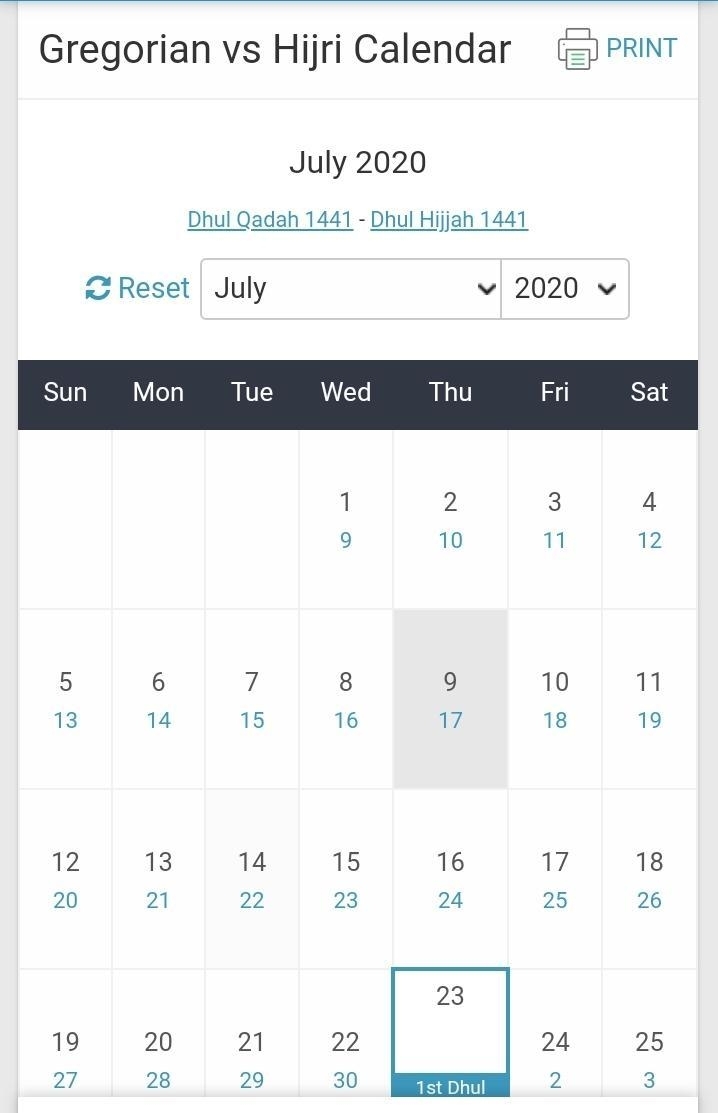This is a detailed screenshot of a calendar interface from either a PC or a phone. At the top, there is a blue-green banner. Below the banner, on a white background with black text, the heading reads "Gregorian vs. Hijri Calendar". Adjacent to this heading is a print icon, also in a bluish-green color.

The calendar displays the month of July 2020, also referenced as "Dhu al-Qi'dah 1441 - Dhu al-Hijjah 1441" in the Islamic Hijri calendar. To the right of the month and year, there is a dropdown menu for selecting different months and years, with "July 2020" currently selected. To the left of this dropdown, there is a "Reset" button, also in the bluish-green color.

The main body of the calendar shows an outlined grid. The days of the week, abbreviated to three letters (Sun, Mon, Tue, Wed, Thu, Fri, Sat), are printed at the top in black. The month begins on a Wednesday, with the 1st of July being a Wednesday, and continues through to Saturday, the 25th of July, which is the last visible date in this screenshot.

Notably, the 9th of July is highlighted in gray. The 23rd of July is enclosed within a box and is marked with the note "1st Tahul".